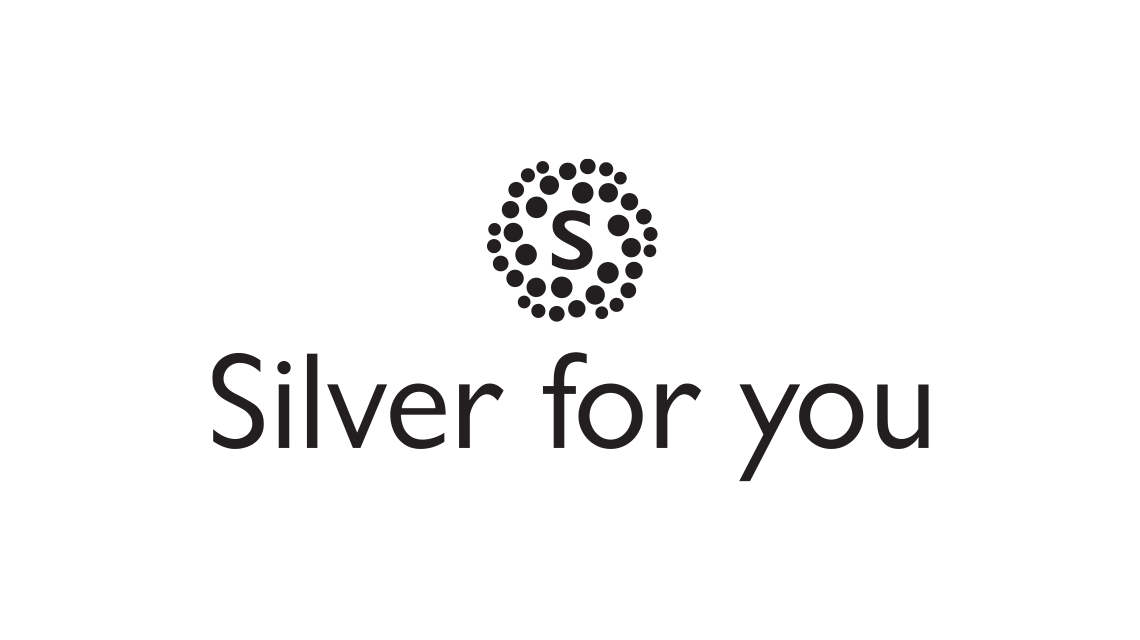The image features a minimalist design set against a completely white background, dominated by a centered, black, swirling logo and some black text. At the heart of the logo, a block-style, capital letter "S" is nestled within a whirlpool of black dots, which vary in size from larger on the left and gradually becoming smaller as they spiral outwards. Below this intricate swirl, at the very center of the image, the phrase "silver for you" is displayed in large, black letters, with the only capitalization occurring at the initial "S" in "silver". The text is devoid of punctuation, adding to the clean and straightforward aesthetic that gives it a professional and polished appearance, akin to a company logo typically found on a business card. The stark contrast between the black elements and the white background highlights the simplicity and elegance of the overall design.